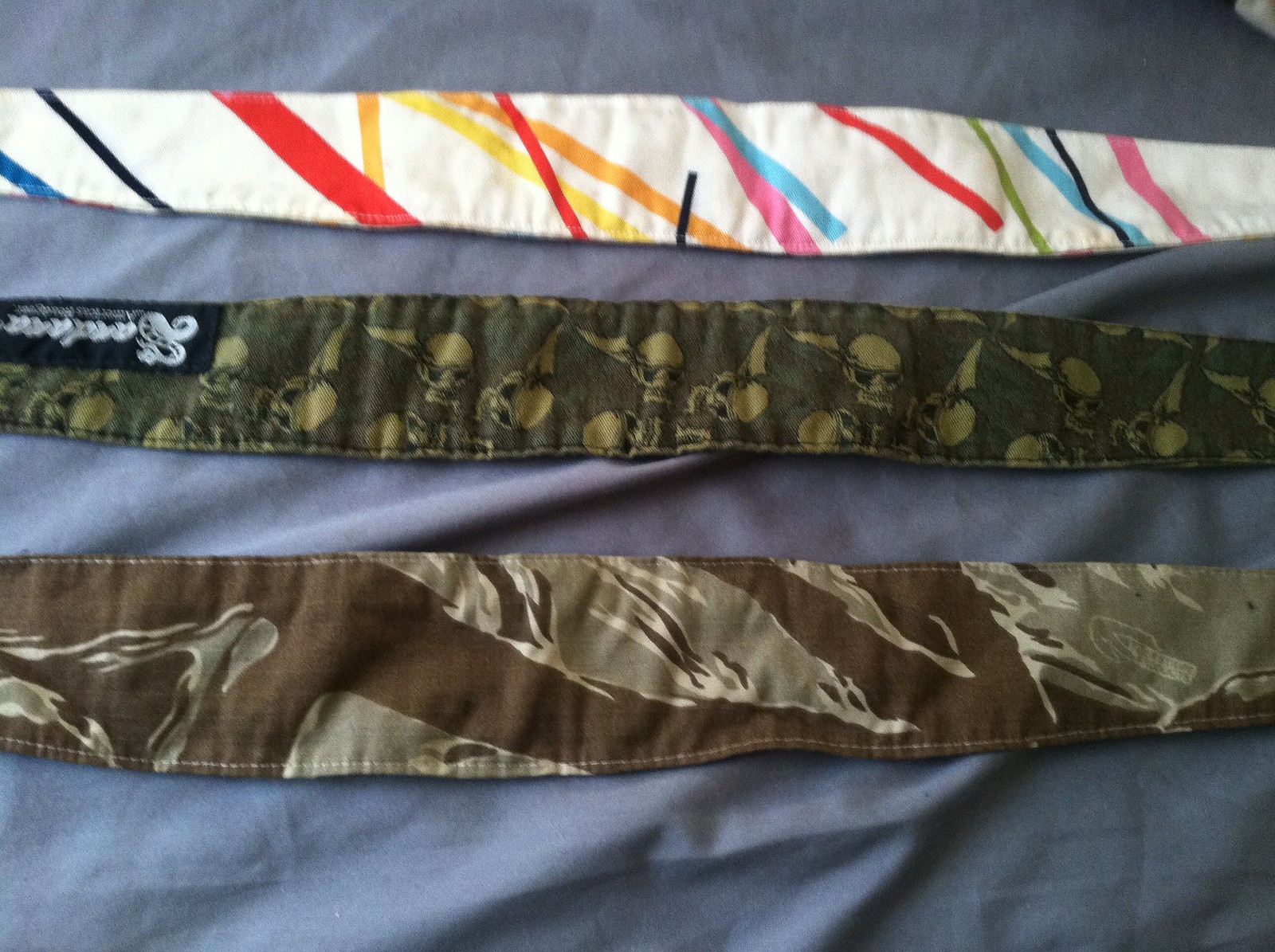The photograph features three bandanas laid horizontally on a wrinkled, greyish-blue sheet. The top bandana has a white background adorned with multi-colored stripes in random orientations, including hues of red, orange, yellow, pink, light blue, dark blue, black, and green. The middle bandana is army green with a dark green background and light green skulls scattered across it. This bandana also has a black tag with white text and a snake symbol on the left side. The bottom bandana displays a desert camouflage pattern with shades of cream, tan, and brown. All three bandanas are broad in the middle, tapering towards the edges.